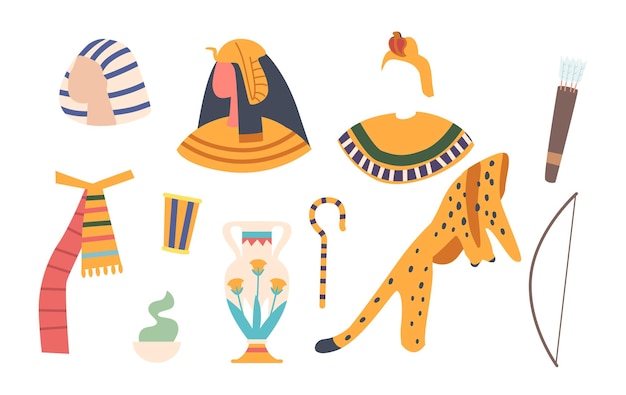The image features two rows of cartoonish vector art, inspired by ancient Egyptian culture, set against a stark white background. In the top row are four distinct items, starting with a flesh-toned head turned to the right, adorned with a beige and blue striped Egyptian headdress. Beside it is another head, colored in a bright reddish-pink skin tone, with a black hairpiece decorated with a dark orange tassel, topped by an orange headdress featuring an ibis. This figure also features an orange and dark orange striped gown. Following this, an empty headdress space above a shoulder drapery adorned with a dark green line and bordered by a dark blue line with white stripes is displayed; the headdress is an orange cap with a cartoon red cobra. The fourth item is a brown quiver of arrows with a light brown band near the bottom. 

The bottom row begins with a multicolored scarf with one tassel in orange with dark green, magenta, and blue stripes, and the other in magenta with dark red stripes. Next are an orange forearm bracer with golden bands at the ends and vertical blue stripes, and a beige bowl emitting green smoke. The following item is a tall beige vase with blue plants and orange flowers emerging from it. The vase features two handles, a blue line around the lip, a red triangle pattern, an orange base with a red stripe. Further along is a bright orange shepherd's crook cane with blue horizontal stripes. Next is a cartoonish jaguar or cheetah pelt, colored in bright orange with dark orange stripes and dark blue spots, capped by a dark blue tail end. Rounding off the collection is a simple brown bow with a matching string. These illustrations appear to be part of a vector art collection available for download.